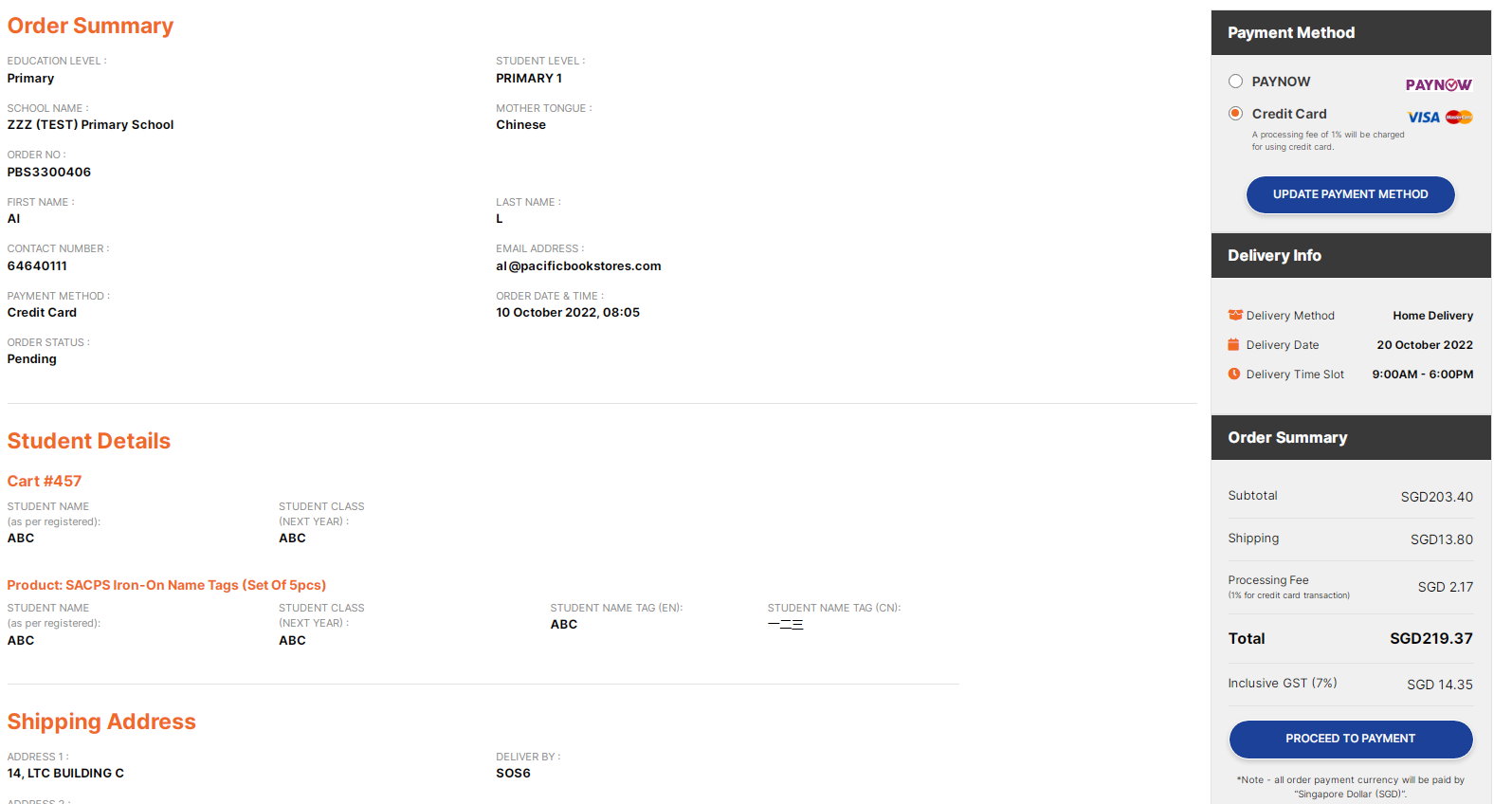The image displays an extensive order summary page, presenting detailed information pertinent to an order that has not yet been completed. The page is designed comprehensively, spanning a wide area to encapsulate all necessary details.

At the top, the order summary specifies the education level as "primary" and the student level as "primary." The school name is marked as "ZZZ Test Primary School," and the mother tongue is indicated as Chinese. The voter number and first name fields have been filled with placeholder text, as well as other relevant sections with dummy data.

A significant portion of the summary includes payment information, indicating that the selected payment method is a credit card. The currency used for the transaction is Singapore Dollars (SGD). The current status of the voter is "pending," and additional details about the student and the shipping address are meticulously outlined too.

On the right pane of the page, the payment method is reiterated as a credit card. At the bottom of this pane, there is a prominent "Proceed to Payment" button. The total amount due is specified as SGD 219.37.

Although it is not entirely clear what the order is for, it appears it might be related to signing up for classes or an online course, based on the context provided.